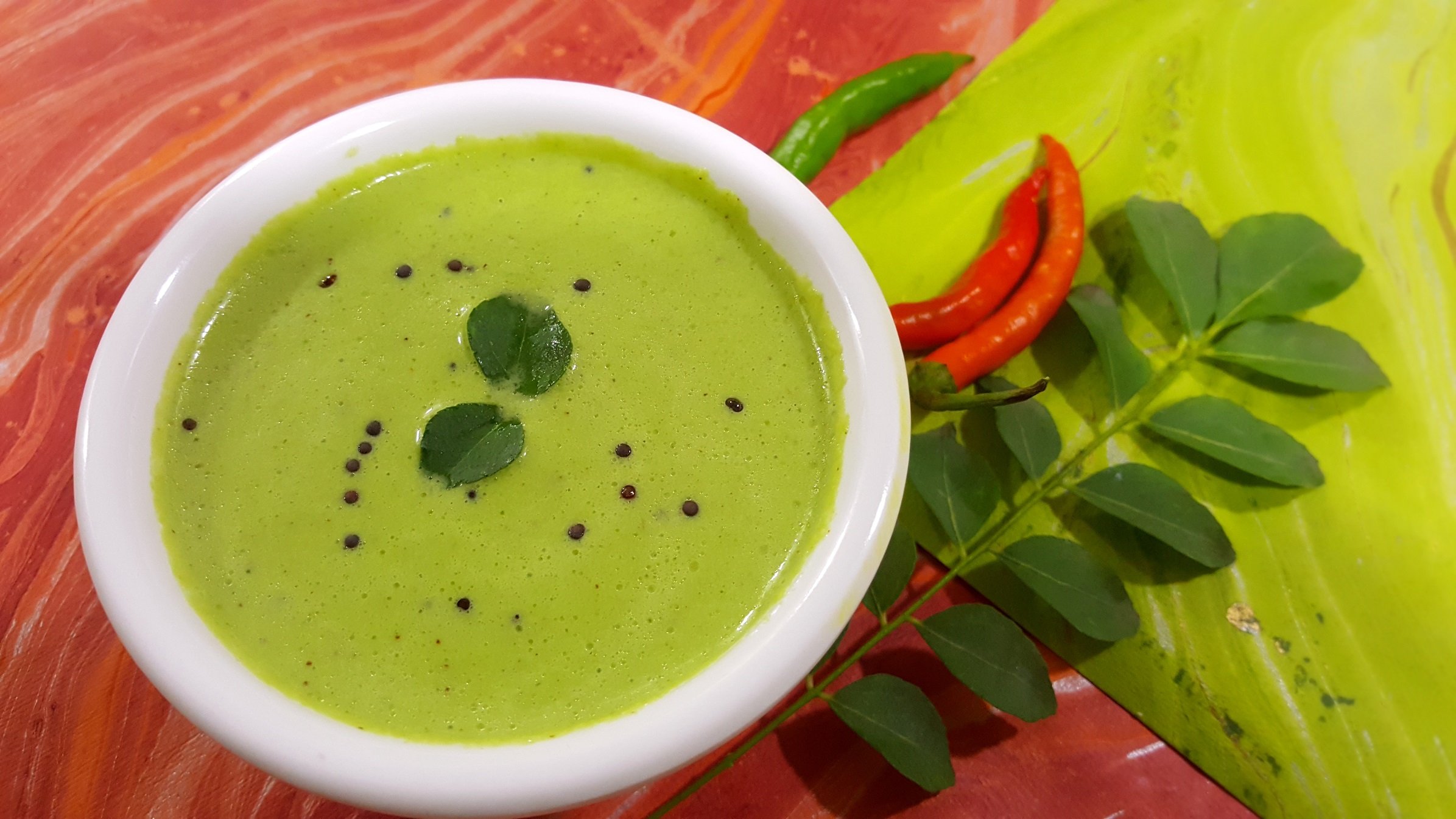The image depicts a close-up view of a small, round, white ceramic bowl filled with a lime-green, pureed soup, which could be a sauce or a creamy soup. The soup is garnished with two leaves that resemble bay leaves floating on its surface, and it is dotted with small black pellets that might be peppercorns. Beside the bowl are a couple of long red chili peppers, likely of the Chinese or Thai variety, and a green stem adorned with dark green leaves, possibly for flavoring or decorative purposes. The items are arranged on a predominantly red, abstract art-inspired painted table that features accents of green and yellow, with a square lime-green mat placed underneath the bowl.